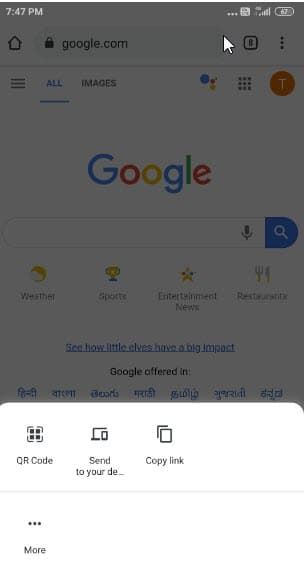A screenshot from a mobile device displaying the Google homepage at 7:47 PM. The screen is slightly grayed out with a prominent white cursor at the top. On the right-hand side of the status bar are icons showing the Wi-Fi connection and battery status, while the left-hand side displays the time. The Google homepage is visible, featuring the Google logo, a search bar, and menu options underneath including 'All', 'Images', 'Weather', 'Sports', 'Entertainment', 'News', and 'Restaurants.' Below the search bar, there is text that reads "See how little elves have a big impact" along with options for language settings. At the bottom of the screen, there's a QR code with options labeled 'Send to your desktop' and 'Copy link,' followed by a three-dot menu and more options. The search bar is empty, with no search query visible.